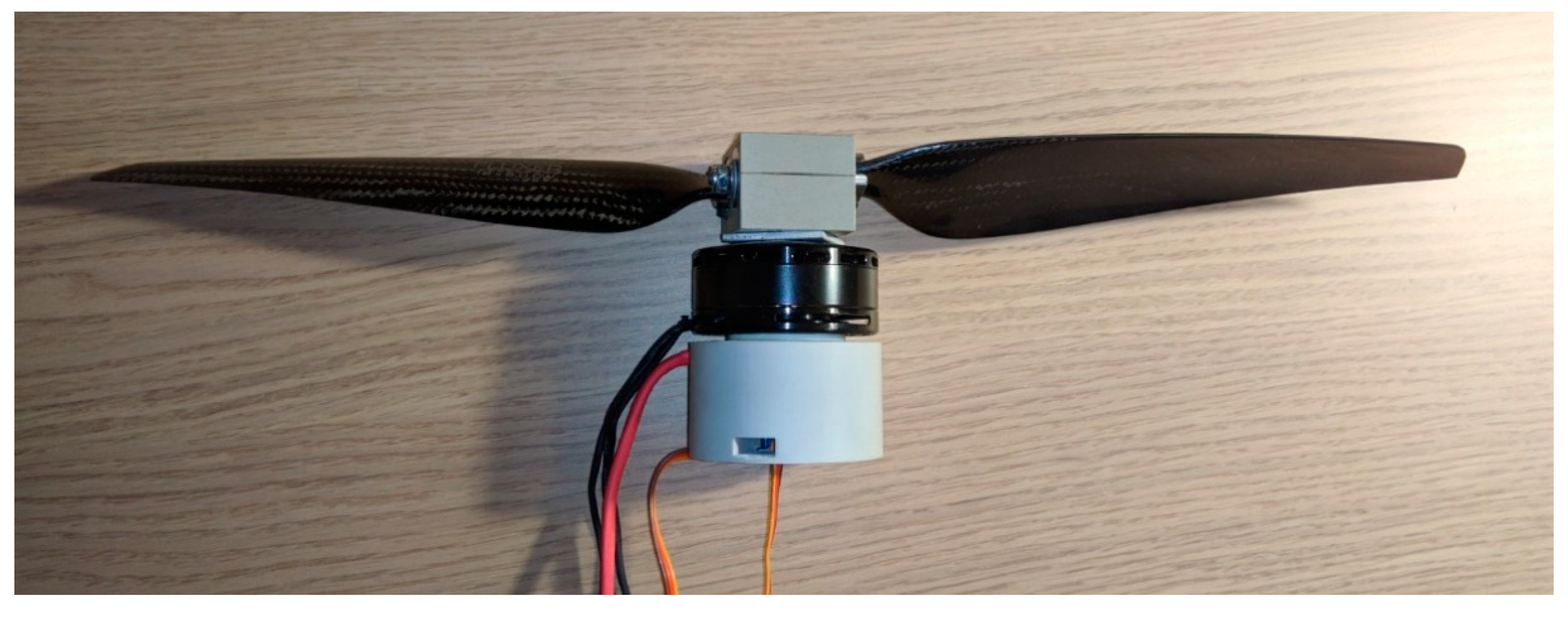The image showcases a mechanical device placed on a light wooden table with varied shading and markings. The device resembles a small rotor or fan with two black blades, each approximately six to eight inches across. These blades are connected to a small, gray, square box by bolts or screws. Beneath this, there's a cylindrical component, with the upper part being black and medium gray, and the lower part transitioning to beige or white. Several electrical wires—two black, one red, and two orange—are prominently visible, extending from the cylindrical part of the device. The photo also reveals a variety of lighting conditions, with some areas brightly illuminated, possibly by a flash, creating contrasting shadows. Overall, the detailed assembly appears to be a compact mechanical or electronic contraption.